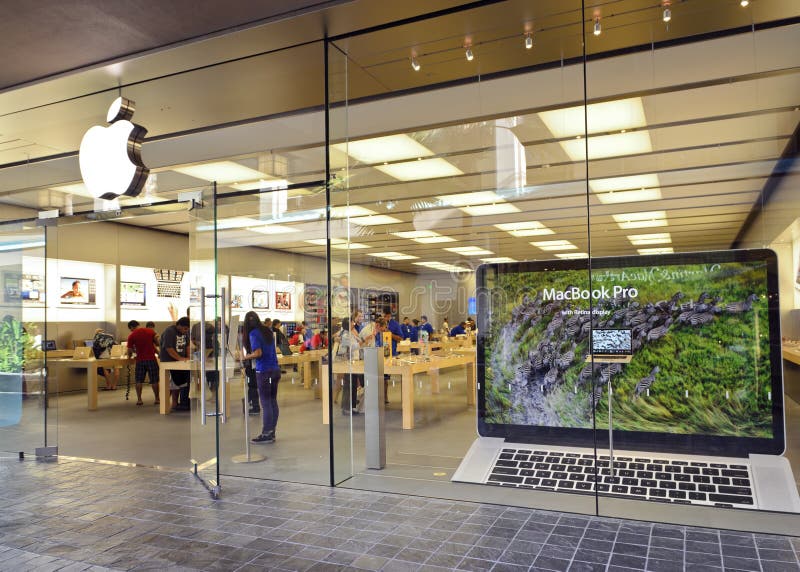A high-tech Apple Store, possibly located in a mall or as a standalone building, is featured in this image. The storefront boasts floor-to-ceiling glass windows, including the doors, offering a completely transparent view into the store's sleek and modern interior. Prominently displayed above the entrance is the iconic Apple logo, rendered in a shiny white-to-silver finish, with its characteristic bite taken out.

Inside, the store is furnished with numerous oak tables, each surrounded by customers exploring the latest Apple products. The left wall is lined with large computer screens, adding to the store's cutting-edge ambiance. A standout feature is a giant MacBook Pro display situated in the lower right corner of the image. The display highlights the MacBook Pro's black keys and sleek silver body, clearly labeled with "MacBook Pro."

Overhead, the ceiling is illuminated by an array of yellowish rectangular lights, which cast gentle reflections on the glass walls, enhancing the store’s bright and inviting atmosphere. This meticulously designed space exemplifies Apple's commitment to innovation and customer experience.